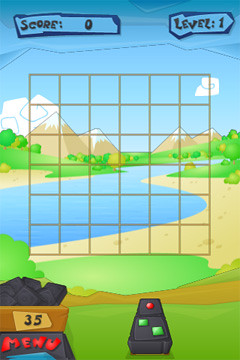The image is a screenshot of a cartoony phone game, likely a puzzle game, featuring a detailed and picturesque landscape. The background showcases a blue sky with a few clouds, green grass, small trees, and four mountain peaks with snowy tops and brown sides. A blue river runs through the scenery, originating from the mountains and flowing off the left side, bordered by sand. Below, the bottom third is covered with green grass and a brown strip running across the middle. 

On the game's interface, the top left corner has a rectangular bar with the score displayed as '0' in black text, and the top right corner features another bar displaying 'Level...1'. The bottom left corner has a small blue box with 'Menu' written in red letters, topped by a wooden box labeled '35' in black text. Nearby, there's a two-piece remote with a red button on the top piece and two green buttons on the bottom piece, positioned diagonally across each corner.

Prominently displayed across the center of the screen is a 7x7 grid, indicating the puzzle aspect of the game.